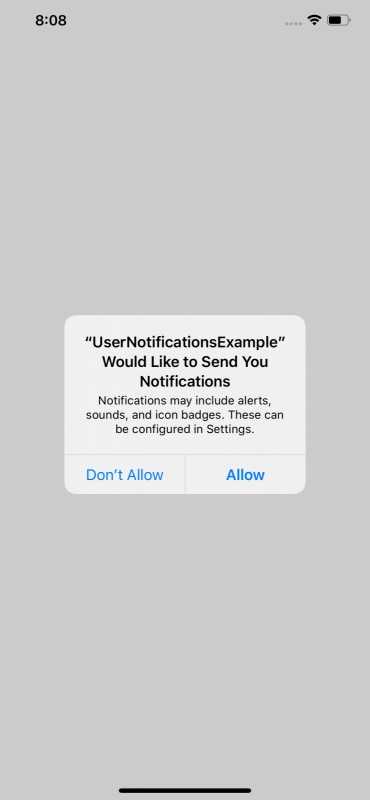A smartphone screenshot displays a predominantly gray background. At the very top, the time is shown on the left at 8:08—its status as a.m. or p.m. is not indicated. On the right are indicators for signal strength, wireless connection, and battery life. The cell signal strength shows no bars, implying no service, while the Wi-Fi signal is strong, denoted by three full bars. The battery icon shows it is over 50% charged but not completely full.

Centrally positioned on the screen is a lighter-colored notification box. The box informs the user, "User Notifications Example would like to send you notifications. Notifications may include alerts, sounds, and icon badges. These can be configured in Settings." Below this message are two buttons; "Don't Allow" on the left in a standard blue hue, and a bolder, more prominent "Allow" button on the right. There are no other elements on the screen aside from this notification box.